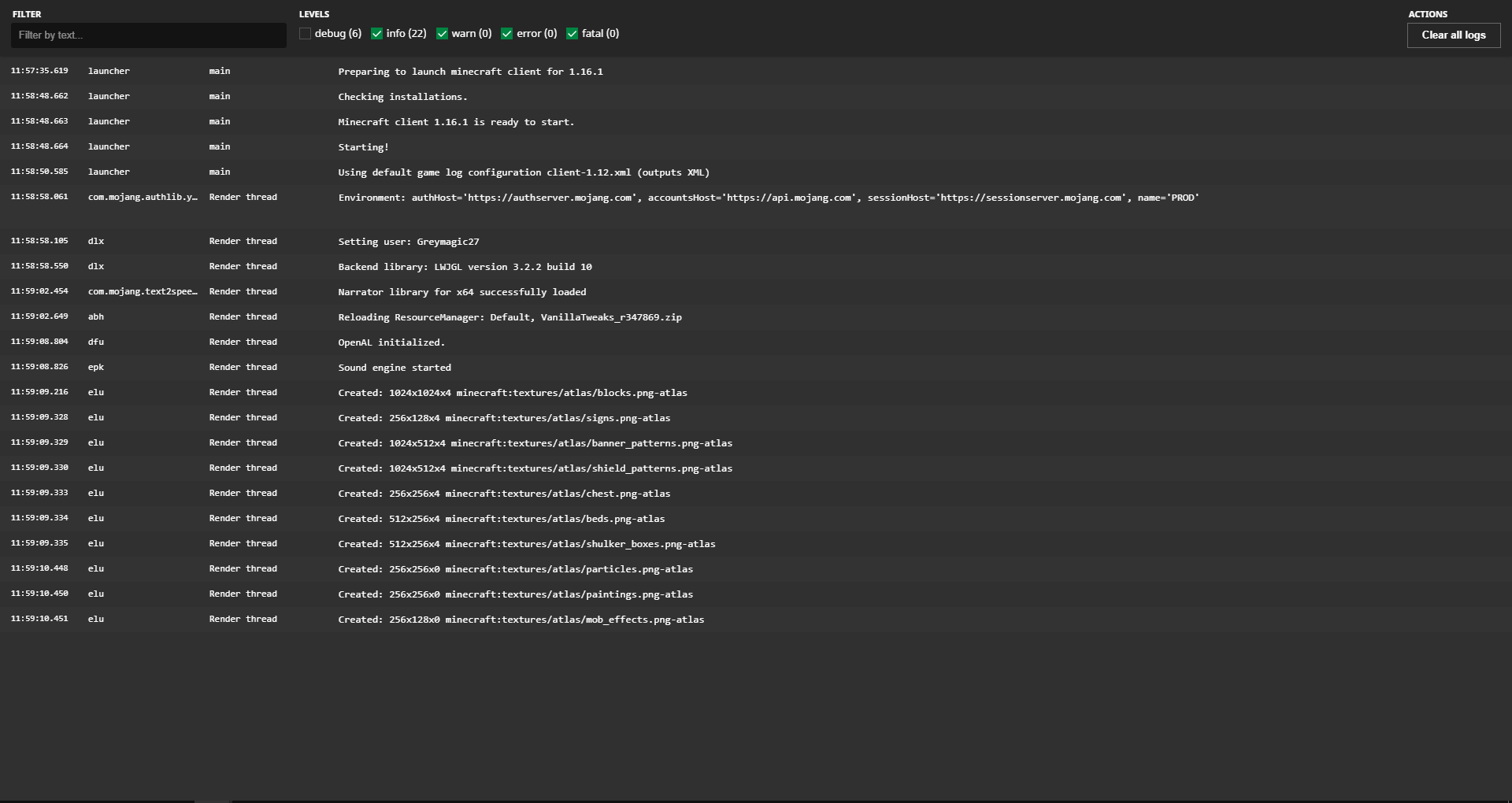A detailed image description based on your caption: 

The image appears to be a screenshot taken from a website interface. The background is predominantly black, which makes the text and other elements stand out. In the top left corner, there is a small text label that reads "Filter." Below this label, there is an even darker input box where users can type in their search criteria or filter terms.

Next to the filter section, there is a column labeled "Levels," with several selectable options listed below it. The first option is unchecked, indicated by an empty square. The subsequent four options are selected, each represented by a green box with a white checkmark inside.

On the top right corner, there is a button labeled "Actions." Directly below this button, there is another option labeled "Clear All," which might be used to reset or remove all selected filters or actions.

The main body of the interface seems to be a structured chart. On the left side of the chart, there is a vertical list that could represent numbers or categories, extending downwards. Adjacent to this list, towards the middle of the chart, there is a column of text that is situated next to blank spaces. This pattern repeats, creating alternating columns of text and blank spaces. 

Each item on the list seems to have a corresponding short sentence or note beside it, providing additional information. This detailed structure suggests the chart is likely used for organizing or sorting data, possibly in a spreadsheet or detailed report format.